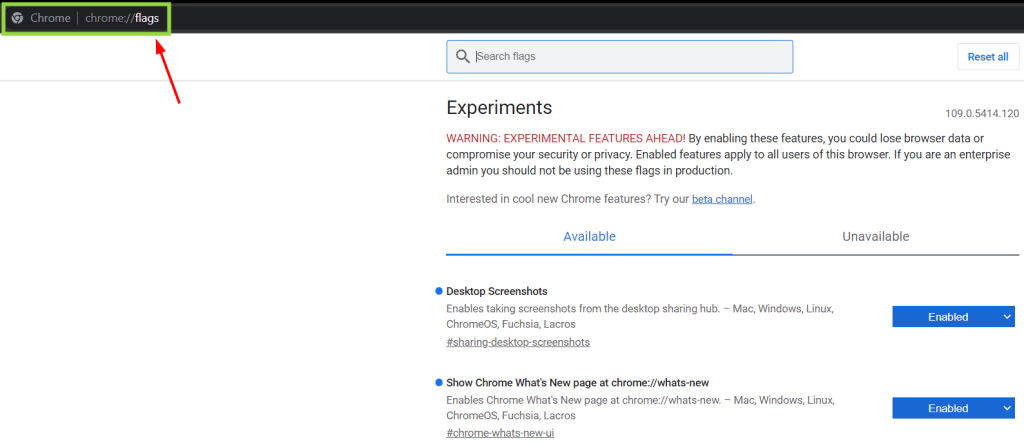The image displays the Chrome browser's experimental features page, accessible via "chrome://flags." The top section has a light green highlight over the browser’s address bar, which reads "chrome://flags" in gray text, except for "flags" which is in white. To the left of the URL, a gray Chrome logo is visible, with a capital "C" in "Chrome" beside it, whereas the "chrome" in the URL is lowercase.

Below the address bar, the page is largely blank on the left side, but the right side features a search function labeled "Search flags." Directly beneath this, a blue "Reset all" button is displayed. The headline reads "Experiments," followed by a red warning: "WARNING: EXPERIMENTAL FEATURES AHEAD!" The warning text reads, "By enabling these features, you could lose browser data or compromise your security or privacy. Enabled features apply to all users of the browser. If you are an enterprise admin, you should not be using these flags in production."

The page suggests, "Interested in new Chrome features? Try our Beta channel," with "Beta channel" underlined in blue, indicating it is a link. Below this, two tabs are labeled "Available" and "Unavailable," with "Available" highlighted in blue, indicating it is currently selected.

Under the "Available" section, the image lists two features: "Desktop Screenshots," with a dropdown menu showing it is "Enabled," and "Show Chrome What's New Page at chrome://whats-new," also "Enabled," both with down-facing carets, indicating they can be expanded or toggled.